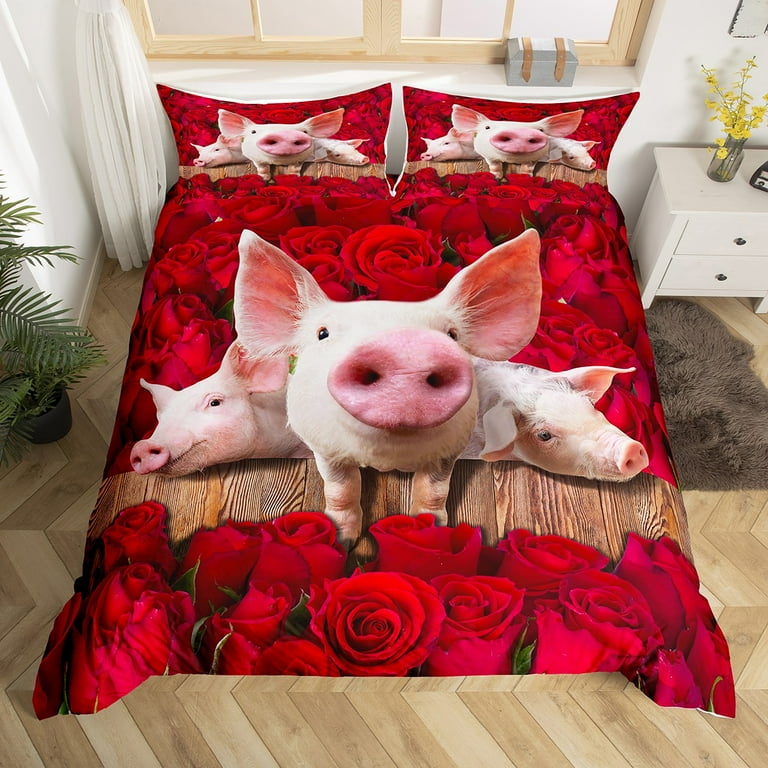The image showcases a charming bedroom with white walls and a large window behind the bed, featuring a silver-colored treasure box with brown straps on its ledge. The room has beautiful light-colored hardwood floors arranged in a herringbone parquet pattern, adding a stylish touch. To the left of the bed, there's a vibrant green potted plant, while to the right, a small end table or coffee table stands beside a cozy blackish fur rug.

The bed itself is the room’s standout attraction, adorned with a striking comforter and pillowcases that depict a vivid and playful design. The bedding features a trio of adorable pigs: one pig staring directly at you with a pink snout and ears almost pressed against the lens, and two pigs either lying down or walking to the side, all set against a lush backdrop of red roses. This whimsical motif gives the bed a playful and eye-catching appeal, as if the image of the pigs was photoshopped onto the fabric. The overall ambiance is warm and inviting, with a small white dresser adorned with a vase of yellow flowers completing the look.